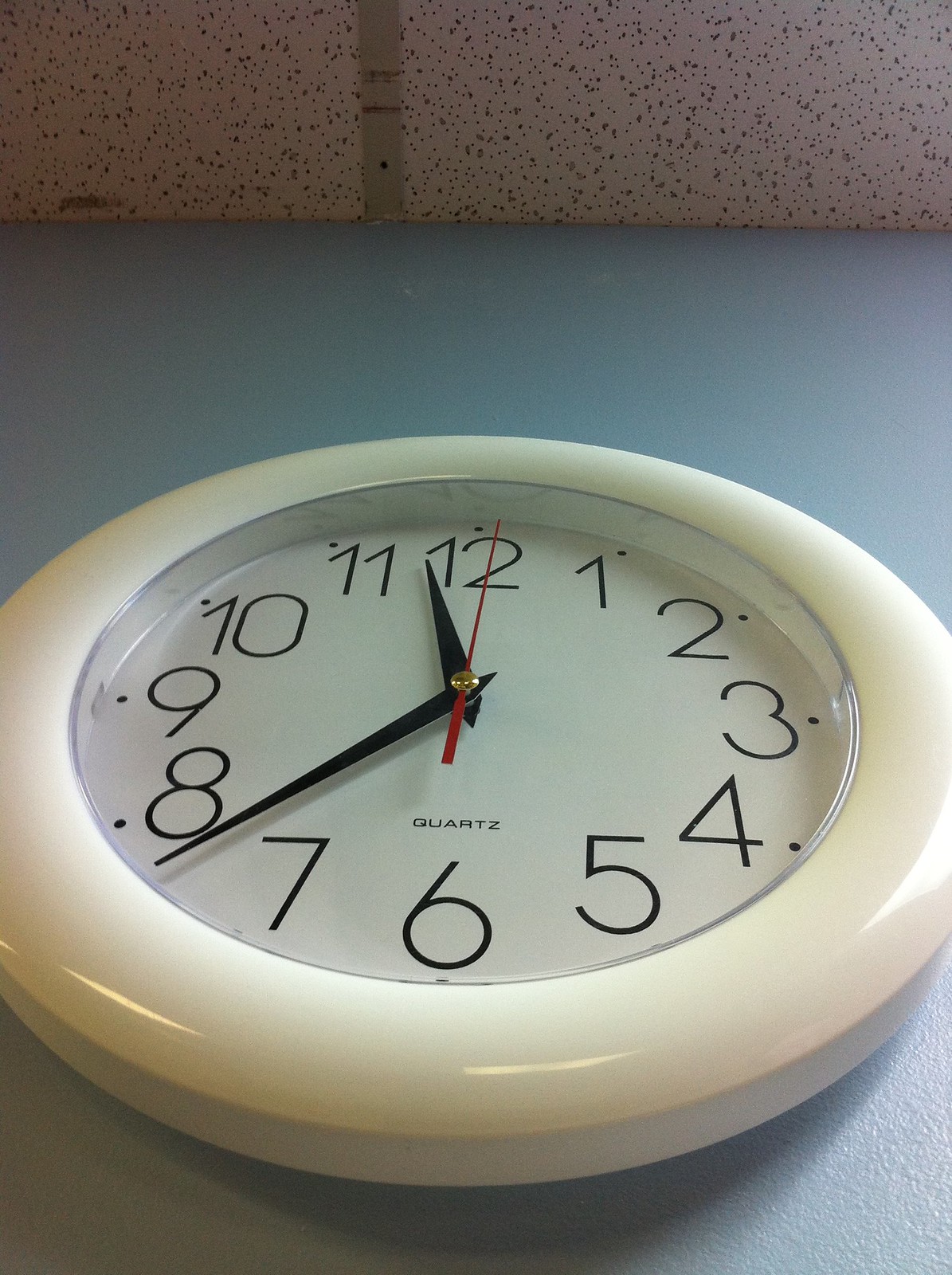This color photograph captures a round white clock mounted on a blue surface, viewed from a low angle. The clock features a thick, creamy-yellow rim with highlights from reflected light. The face of the clock is white, with black numbers ranging from 1 to 12. The clock has two black hands: the minute hand points to 8, while the hour hand is positioned between 11 and 12. Additionally, a small red second hand is pointing precisely at 12. A shadow is cast beneath the clock, enhancing its three-dimensional appearance. At the very top of the image, grey bricks are visible, suggesting the clock is likely attached to a wall. The word "Quartz" is printed in black just above the number 6 on the clock face.